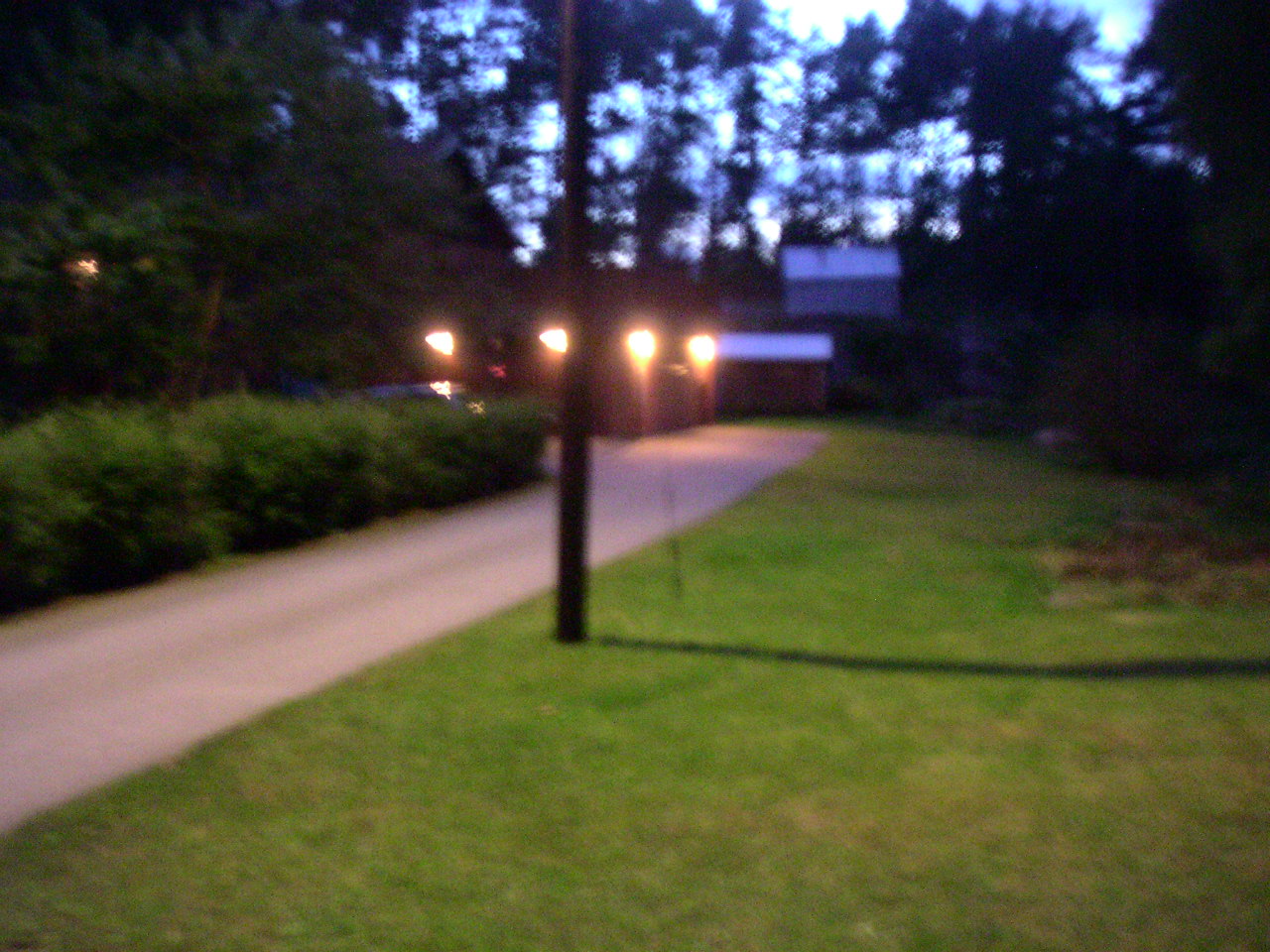The image depicts a blurry photograph taken at dusk, either very early dawn or close to sunset, capturing an outdoor area. Dominating the left side, a dirt or cement walkway runs diagonally through the scene, with low green shrubs and an open grassy field to its right. In the dim light, the general atmosphere appears dark, contributing to the photograph's overall blur. In the background, tall, indistinct trees frame the scene, their placement uncertain due to the shadows. Four orange fluorescent lights attached to a small, indistinct building with a white roof cast their glow. The driveway leads up to this structure, while beyond it, another white-roofed building is faintly visible. The sky appears blue, purple, and white, accentuating the silhouettes of the blurred pine trees in the upper parts of the image. Overall, the photograph hints at a residential area, characterized by its indistinct and out-of-focus elements.